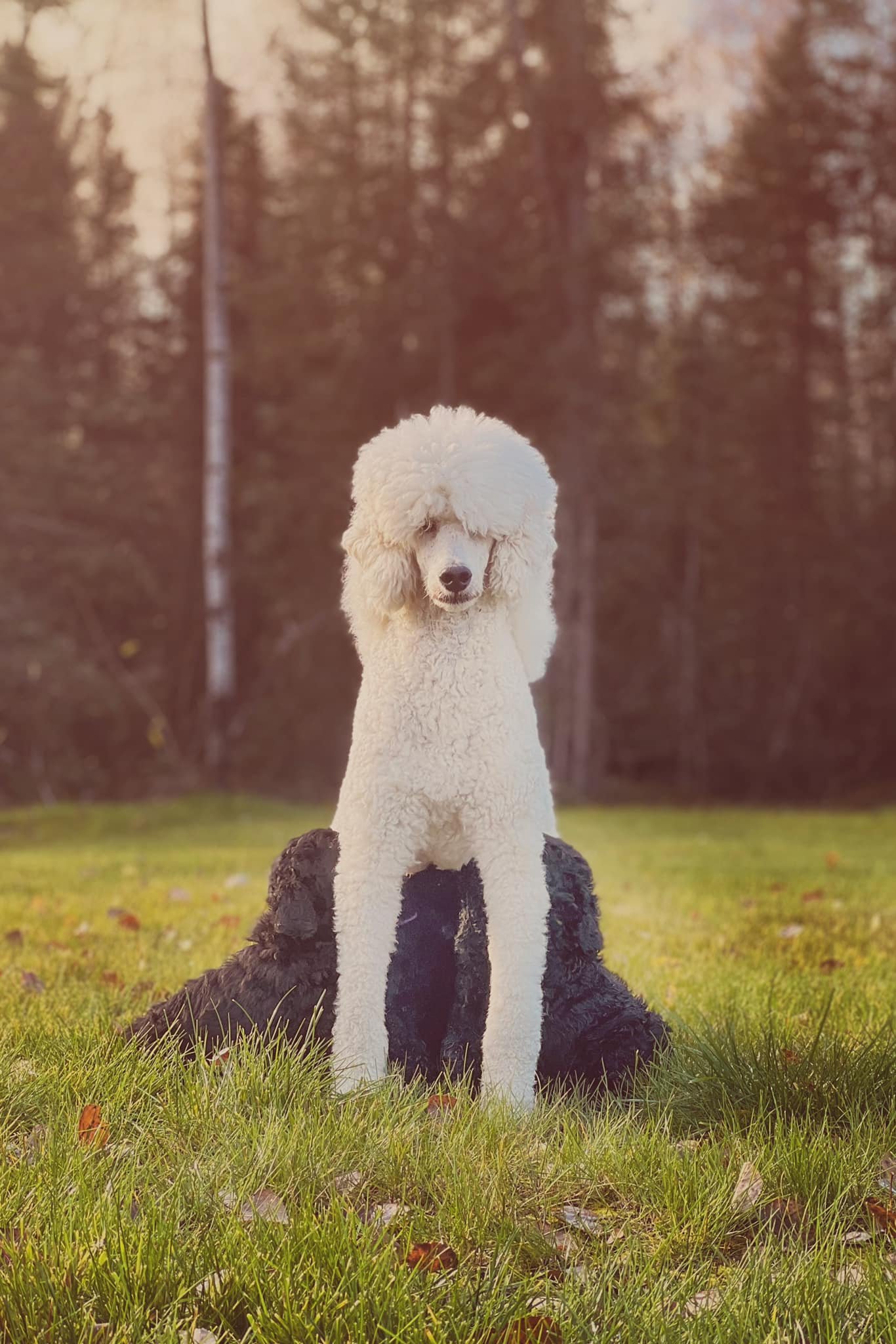In this captivating image, we observe a fluffy, white dog from a frontal viewpoint, nestled amidst a ground lush with green grass and a few scattered leaves. The dog sits majestically, displaying a soft brown nose and endearing white face, its two paws resting gently over what appears to be a group of small, dark brown or black puppies underneath it. The puppies are huddled close, creating a touching scene of canine affection. Framing the dog in the background are towering trees adorned with green leaves, through which patches of a gray sky subtly peep.